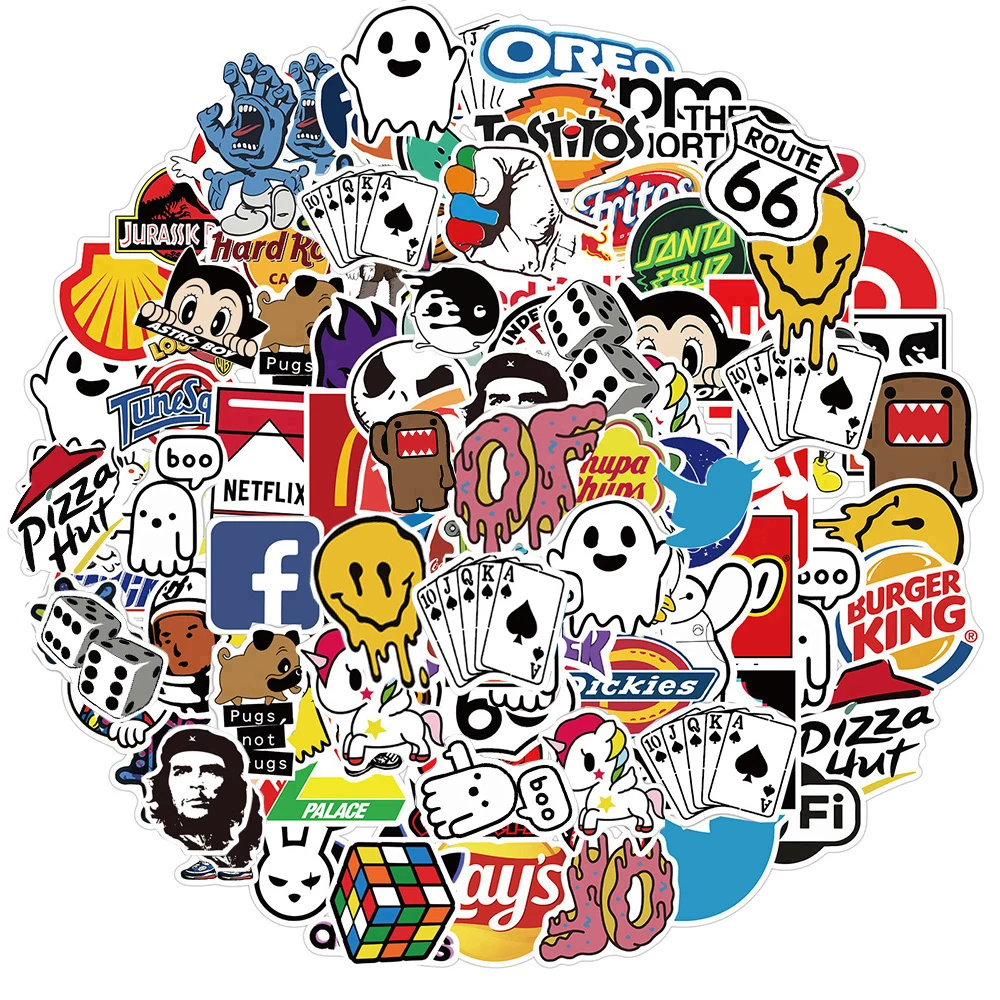The image is a vibrant and meticulously arranged collage of familiar and popular logos, all combined into a circular formation against a white background. At the very center of this circle is the 'oh F' logo in a donut frosting color. Surrounding it are an array of well-known logos: the Route 66 sign with white background and black letters is located at the top right, while the Burger King logo featuring the iconic orange bun and red letters sits on the right side. At the very bottom, the Lay's potato chip logo is prominently displayed next to a Rubik's Cube with its distinct yellow, white, red, and blue faces. Anchoring the left side is the Pizza Hut logo, and the top of the circle features the Oreo logo.

The assortment also includes logos of brands like Tostitos, Hard Rock Cafe, Facebook, Netflix, McDonald's, Lego, Shell, Jurassic Park, and various stickers and decals like a cartoon ghost, a unicorn, dogs, and poker hand showing a straight flush. This collage showcases a diverse palette of colors, primarily white and black, but punctuated with vivid reds, yellows, and blues, reflecting the unique identities of each logo.